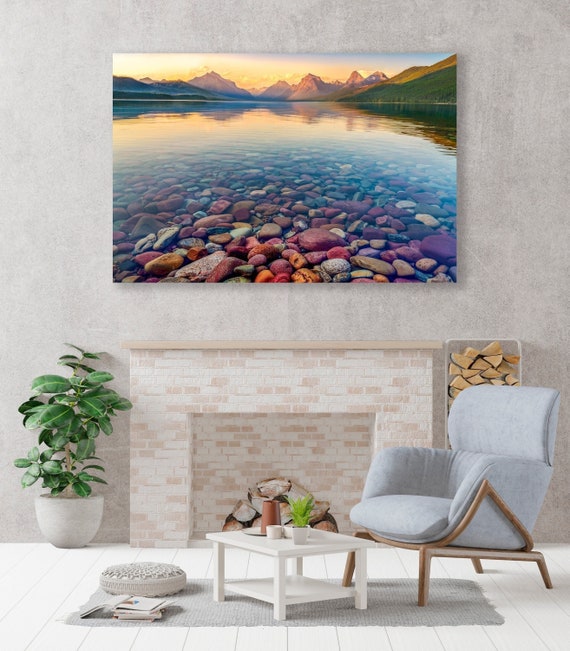The image portrays an intricately designed living space, possibly a living room or a display area within a store. The focal point is a sophisticated, tiled fireplace situated centrally in the room. While it features logs, the fireplace appears non-functional and serves mainly for display purposes, lacking a visible exhaust system. Above the fireplace hangs a vibrant painting of a river nestled amongst mountains, with an array of colors including reds, blues, greens, pinks, oranges, and purples, contrasted against a pale pink and white sky. This artwork starkly contrasts the room's otherwise light and subdued palette of whites, pastels, and light grays.

In front of the fireplace is a cozy setting with a low-seated, grayish-blue chair placed adjacent to a modern white coffee table, which holds a coffee mug and a small plant. The floor features a mix of tiles and a textured rug, upon which a few books are scattered. Wooden logs are neatly stacked to the right side of the fireplace, enhancing the rustic ambiance, while a taller plant flanks the left side, adding a touch of greenery. Near the fireplace, a larger plant stands at roughly the same height, contributing to the room's balanced aesthetic. The overall setting is one of modern elegance, accentuated by carefully curated details and a harmonious blend of colors and textures.